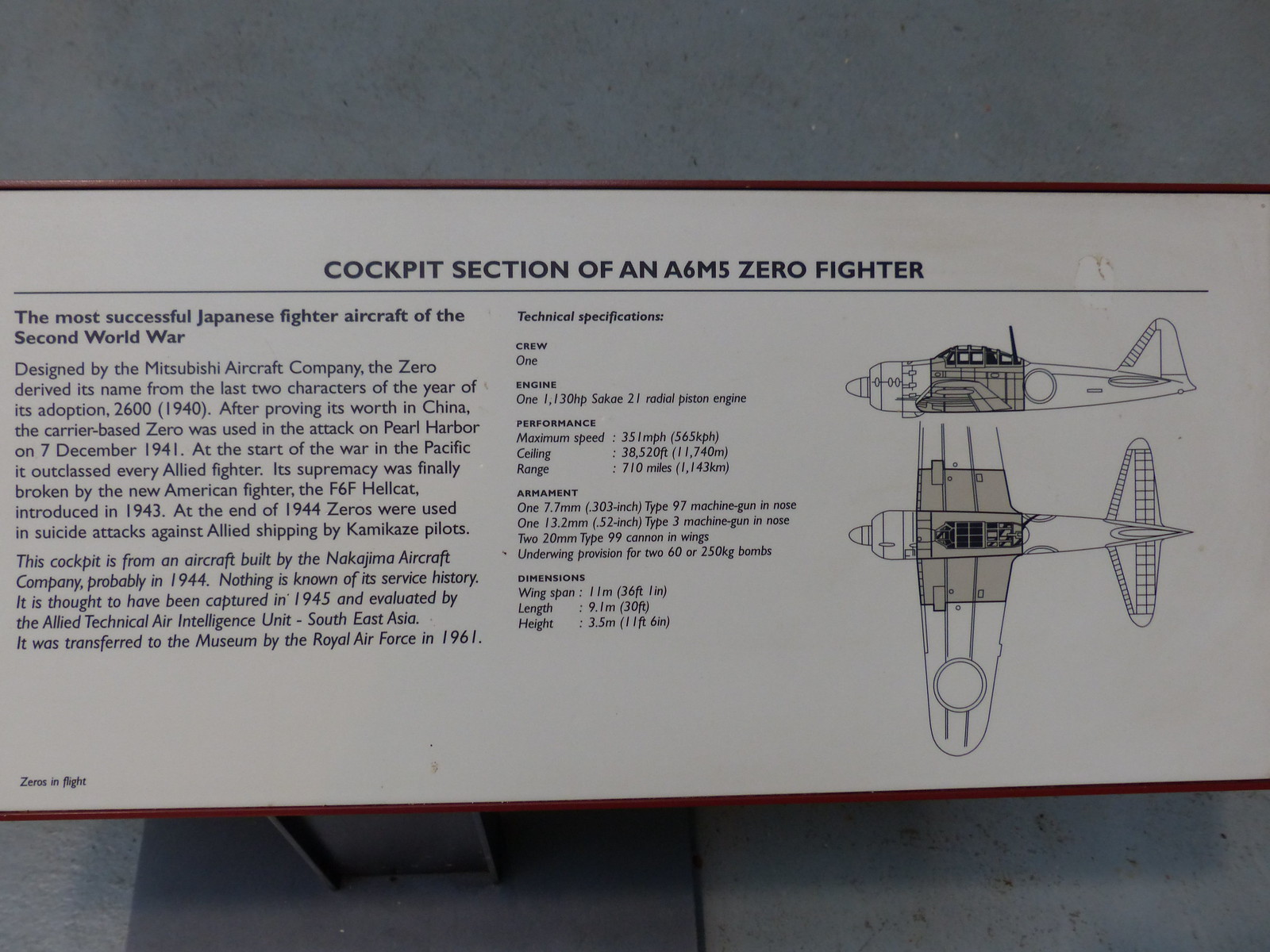This detailed image depicts an informational plaque mounted on a gray column with a base, possibly standing on a concrete floor. The plaque, white with a dark red outline and black uppercase text across the top, is titled "COCKPIT SECTION OF AN A6M5 ZERO FIGHTER." Below the title is a long black horizontal line. On the left side, the plaque contains the heading "THE MOST SUCCESSFUL JAPANESE FIGHTER AIRCRAFT OF THE SECOND WORLD WAR," followed by a couple of paragraphs providing historical context. These paragraphs explain that the aircraft was designed by the Mitsubishi Aircraft Company and was adopted in the year 2600. The A6M5 Zero proved its effectiveness in China before participating in the attack on Pearl Harbor on December 7, 1941. Initially outclassing all Allied fighters in the Pacific, its supremacy was eventually challenged by the introduction of the American F6F Hellcat in 1943. By the end of 1944, the Zero was employed in kamikaze attacks against Allied ships. The cockpit on display is from a Nakajima Aircraft Company-built plane, likely from 1944, thought to have been captured in 1945 and evaluated by the Allied Technical Air Intelligence Unit Southeast Asia. It was later transferred to the museum by the Royal Air Force in 1961.

On the right side of the plaque, the section title, "TECHNICAL SPECIFICATIONS," is written in italicized font. It is followed by detailed headers and lists outlining the aircraft's crew, engine, performance, armament, and dimensions. Adjacent to the text, black-and-white illustrations provide top and side views of the A6M5 Zero fighter, offering a visual reference to complement the detailed written information.